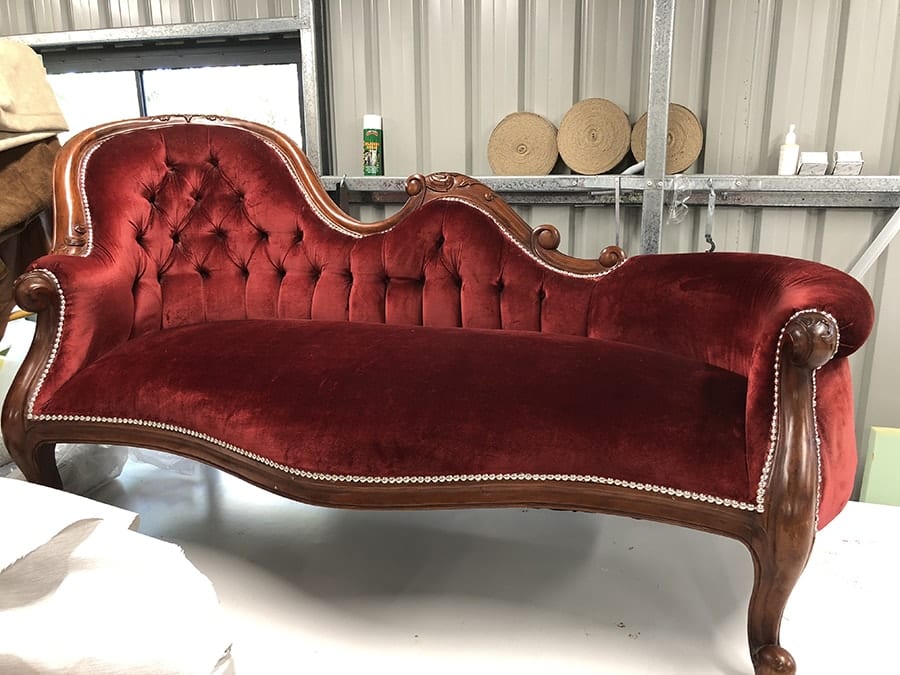The image depicts a large, antique-style red velvet loveseat positioned centrally in what appears to be a garage or shed with sheet metal walls. The sofa, which is taller on the left side and gradually lowers towards the right, features a distinct, curved backrest adorned with tiny circular notches. It is framed by dark brown wood trim, embellished with beaded gems and intricate white patterns, and supported by wooden legs. Above and behind the loveseat, there are metal shelves holding a variety of items, including yarn circles, spray cans, and napkins. In the top left corner, double doors are visible, potentially providing entry to the space. The floor is a stark white concrete, with a shadow cast beneath the couch, and additional miscellaneous objects, such as blankets, can be seen in the background.